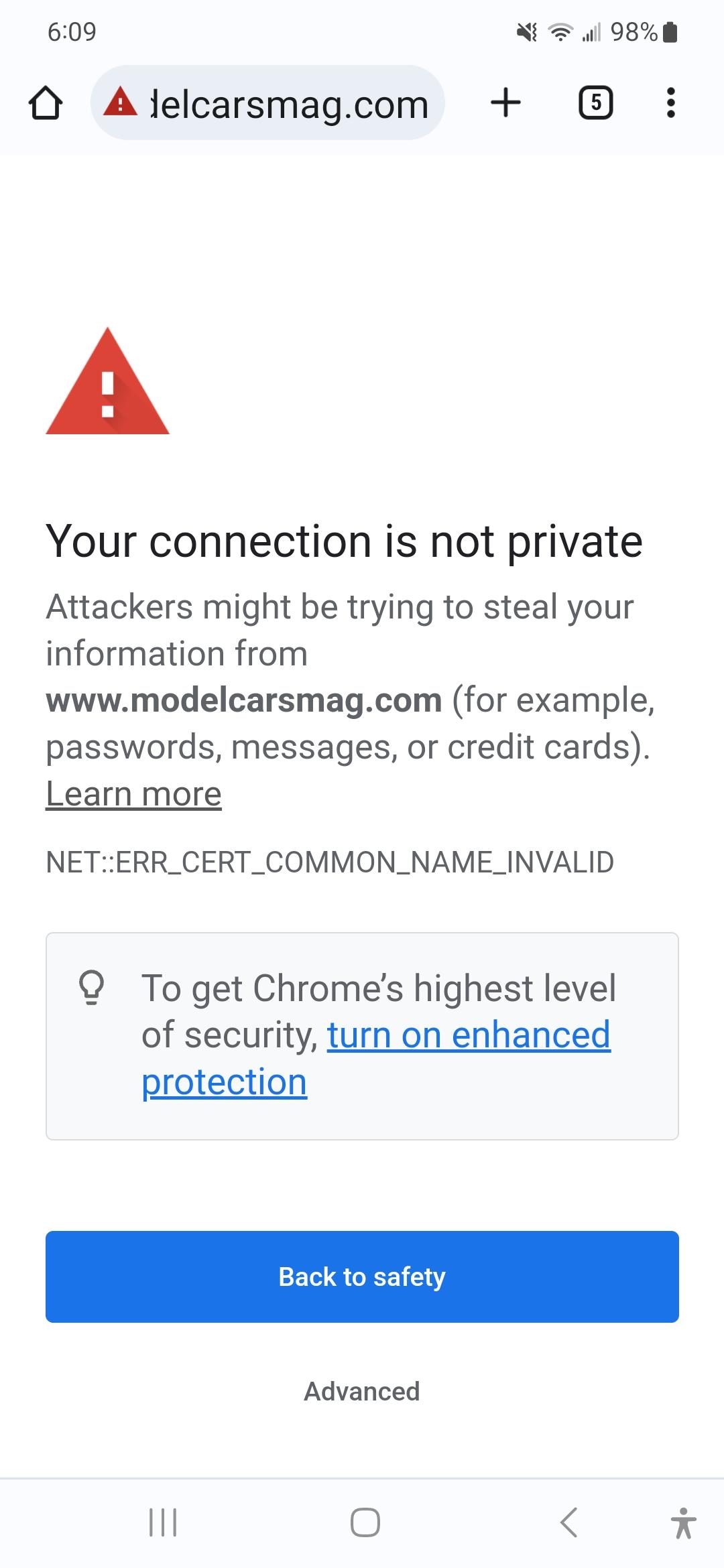A detailed screenshot captures an Android device's warning message about an insecure connection to modelcarsmag.com. The prominent error message reads, "Your connection is not private," warning that attackers may be trying to steal information such as passwords or credit card details. This alert suggests users learn more about the possible threat. Displayed within the Google Chrome browser, the message encourages users to get the highest level of security by turning on enhanced protection, with this suggestion emphasized in bold text. A blue button labeled "Back to safety" and an "Advanced" option offer ways to navigate away from the potential threat.

At the top of the screen, the browser's URL bar includes a red flag symbol next to the web address, further indicating security concerns. The page also features a red triangle with an exclamation point icon, signifying trouble. The user has five tabs open, visible through the tab bar's layout displaying a plus sign and a three-dot menu for additional options. The current time shown is 6:09, and the device's status bar includes icons for Wi-Fi connectivity and a battery indicator at 98%.

The entire interface, predominantly white, underscores the critical nature of the security warning. This screenshot clearly illustrates an attempt to access a potentially unsafe website, highlighting various browser and device elements that alert users to the associated risks.